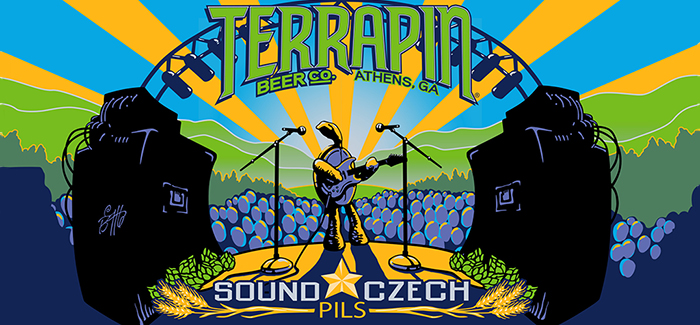The poster features bold green letters at the top reading "Terrapin," with smaller green letters underneath stating, "Beer Company, Athens, Georgia." The background showcases a blue sky with alternating yellow and blue sunbeam stripes radiating outward from a Sun that's dipped below a green mountain range. Below the mountains, a tree line and a crowd represented by unmarked light blue ovals create a bustling atmosphere. Center-stage stands an anthropomorphic turtle with a round shell torso, playing a large guitar that faces away from the audience. Below the turtle, the text reads "Sound Czech" with a yellow star between the words, followed by "PILS." The stage is flanked by two large black speakers, grounding the scene in a musical setting. The overall artwork captures a lively concert moment, promoting the Terrapin Beer Company with vivid, playful imagery.